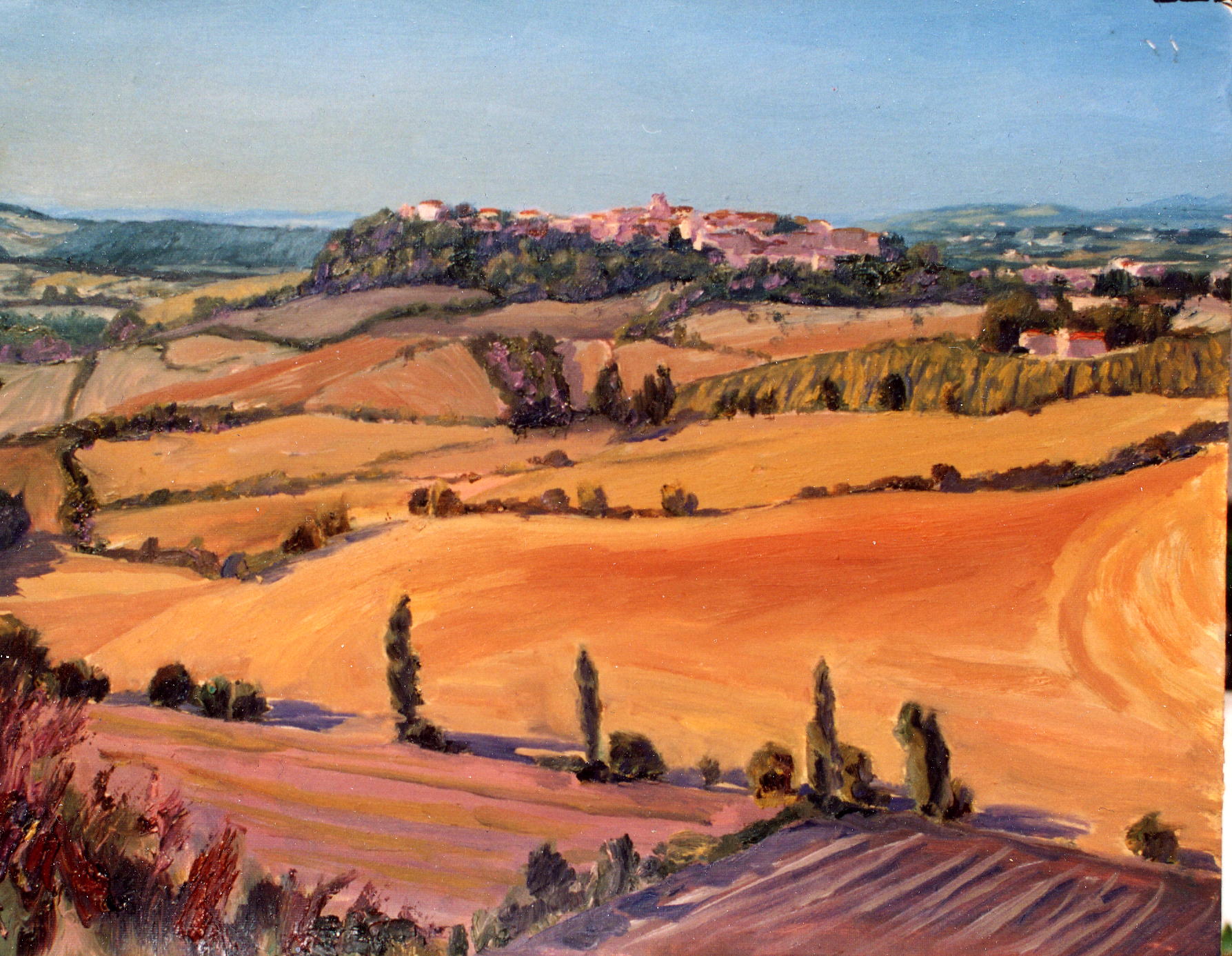The image depicts an impressionistic watercolor painting of a varied outdoor scene bathed in a warm, golden hue with touches of pink. In the distant background, the scene opens up to a clear, light blue sky that meets a greenish-blue mountain range. Below, a vibrant green hilltop crowned with a brownish cluster of indistinct buildings ushers in rolling hills varying in shape and height, painted in brownish-green tones. Moving to the foreground, the colors shift to warmer orange tones covering the ground. 

On the left edge, a road meanders curvilinearly, flanked by lush green plants and orange and pink flowers. The road snakes through a landscape dotted with clusters of green trees and expansive brown fields, lending a sense of a vast, open countryside. Farmland occupies the forefront, giving way to even more brown rolling hills that are sparsely populated by tiny scattered trees. Overall, the scene is a harmonious blend of natural elements depicted in soft, muted colors, evoking the serenity and vastness of a rural outdoor vista.